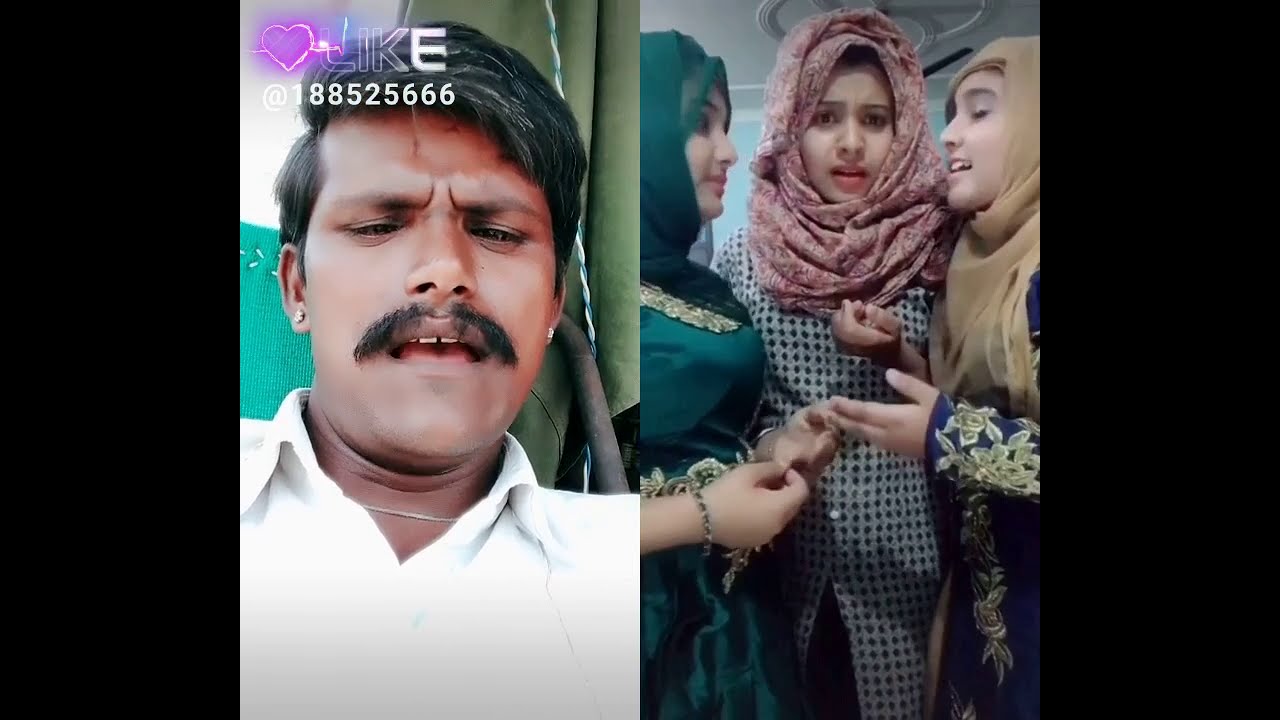The image features two separate photographs side by side, flanked by black rectangles on both the left and right edges. The left photograph is a close-up of an dark-skinned Indian man with black hair streaked with gray, and a mustache. He has a silver chain necklace and stud earrings. The man's expression is one of consternation, with furrowed brows and an open mouth, as though he is speaking. He is dressed in a white button-up polo shirt. Above his face is a heart graphic with the word "LIKE" beside it, followed by the text "1-88-525-666" in white font.

The right photograph shows three South Asian women standing in a circle, appearing to converse or sing, with one looking directly at the camera while the other two face each other. The first woman on the left wears a green headdress and matching outfit. The woman in the middle dons a pinkish headdress and a checkered jacket. The third woman on the right is dressed in a blue floral-patterned outfit with a tan headdress. The diverse elements in these images include various shades of black, white, gray, pink, purple, green, gold, red, yellow, and brown.